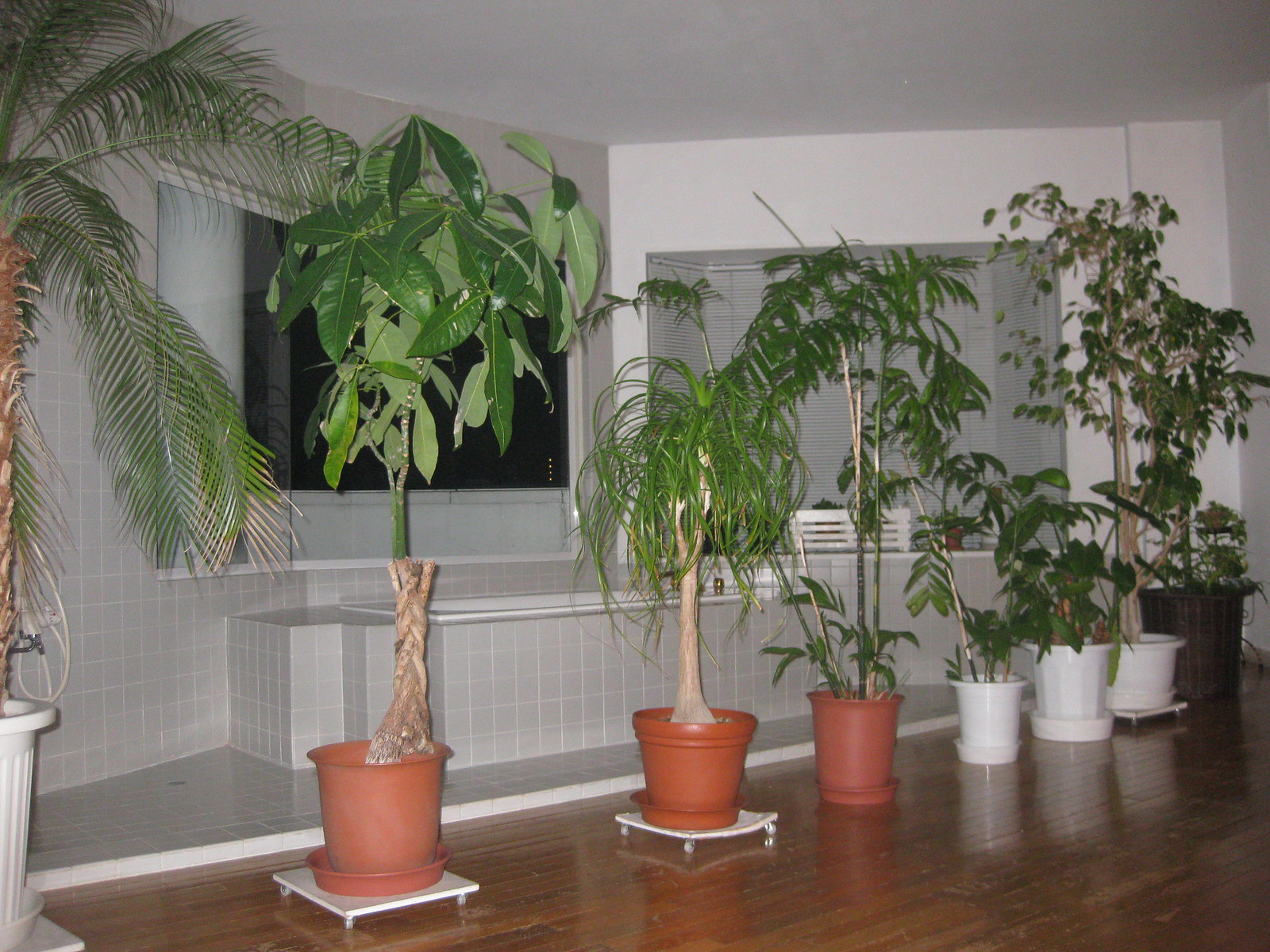This photograph captures a room in a house, possibly a bathroom, featuring an array of indoor plants as its focal point. The back wall, painted in a grayish hue, serves as a contrasting backdrop to the lush greenery. The left-hand side of the image showcases a gray tiled area with a gray tiled bench in front, suggesting a potential spa-like environment. The dark brown wood floor stretches from the bottom left to the bottom right corner of the frame. Arranged diagonally from the bottom left to the top right on the wood floor is a row of eight potted plants.

The pots vary in color: most are white, some are orange, and one at the far right end is black and the largest of the bunch. These pots, likely made of plastic, house various trees and shrubs, including a noticeable small palm tree and large ferns or tropical plants. There appears to be some ambiguity regarding an additional object in the background, which could be a giant TV or a large mirror reflecting the plants. The dark edges around the screen suggest that the photograph might have been taken with a flash. The ambient lighting seems dim, accentuating the plants' vibrant forms against the subdued tones of the room's decor.